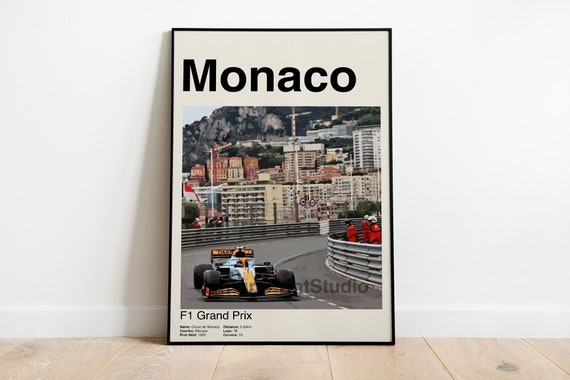A thin black-framed poster, displayed in landscape orientation, is leaning against a white wall on a light brown wooden floor consisting of various planks. The poster's top section features the word "Monaco" in large black letters on a white background. Below that, an action-packed racing scene unfolds: a yellow and black race car with black tires speeds around a curve, encircled by silver guardrails, with a detailed cityscape of reddish, yellow, and white buildings in the background. Lush green trees and a blue sky add vibrancy to the upper left corner of the image. On the right side, a dedicated pit stop crew in bright orange jumpsuits and white helmets attends to the race. The dark grey and light grey street, with its dotted white lines, enhances the sense of motion. At the bottom left, "F1 Grand Prix" is printed in black on a white background, alongside additional unreadable text. The entire scene is bordered by a white margin, framed by a thin black edge. The shadow of the leaning poster adds depth to the overall composition.